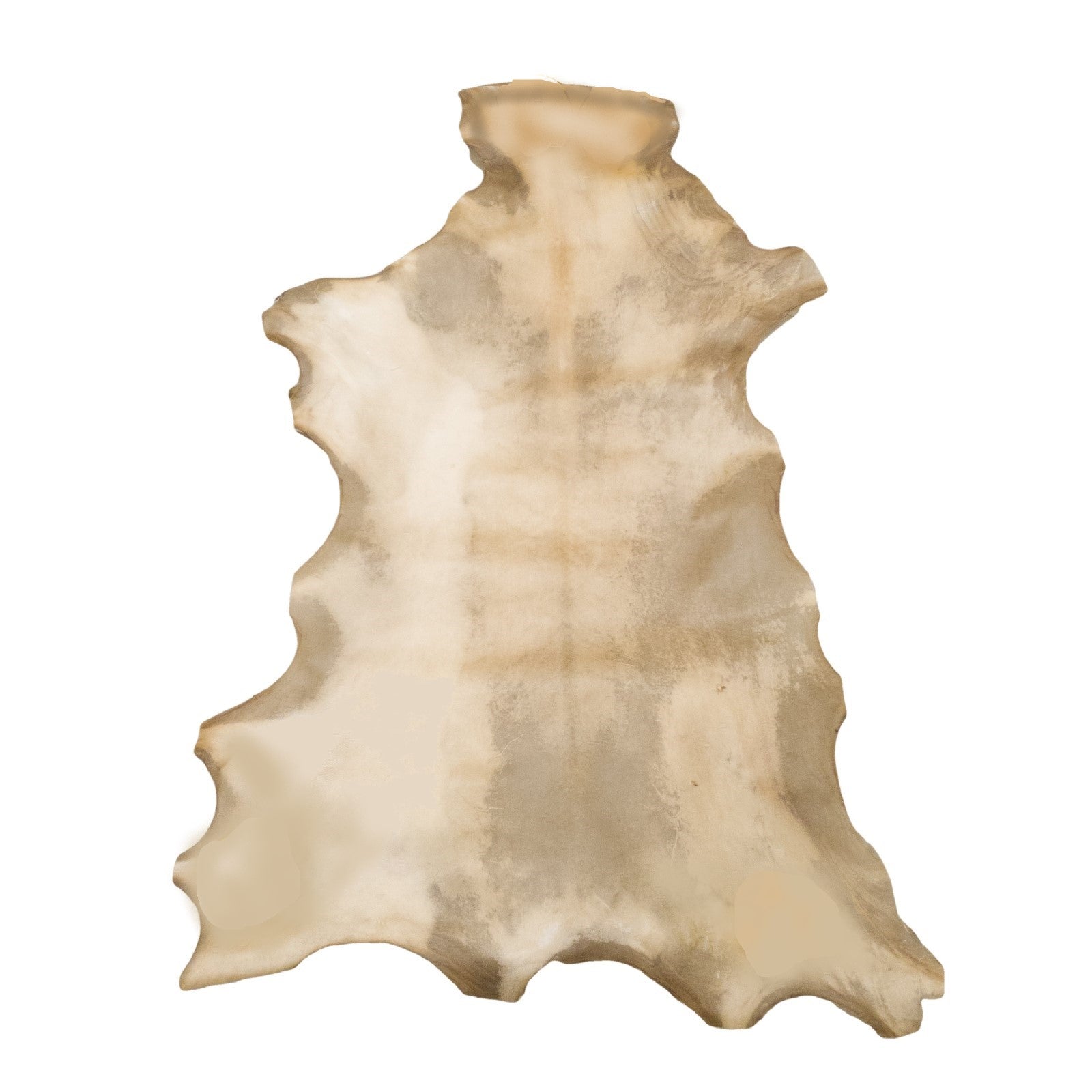The image depicts a piece of animal pelt lain on a completely white background. The hide has a distinctive irregular shape, narrowing at the top and broadening out towards the bottom, somewhat resembling a crudely triangular form. Its surface is smooth and devoid of fur, potentially indicating mummification, with a texture and coloration suggesting it might have once been used for writing or warmth. The pelt is predominantly cream and tan in color with some lighter and darker blotchy spots. Down the center, darker lines run perpendicular to the former location of the animal's spine, suggesting where there may have been natural folds or rolls in the skin. The edges are jagged and uneven, giving it a rough, scalloped appearance.